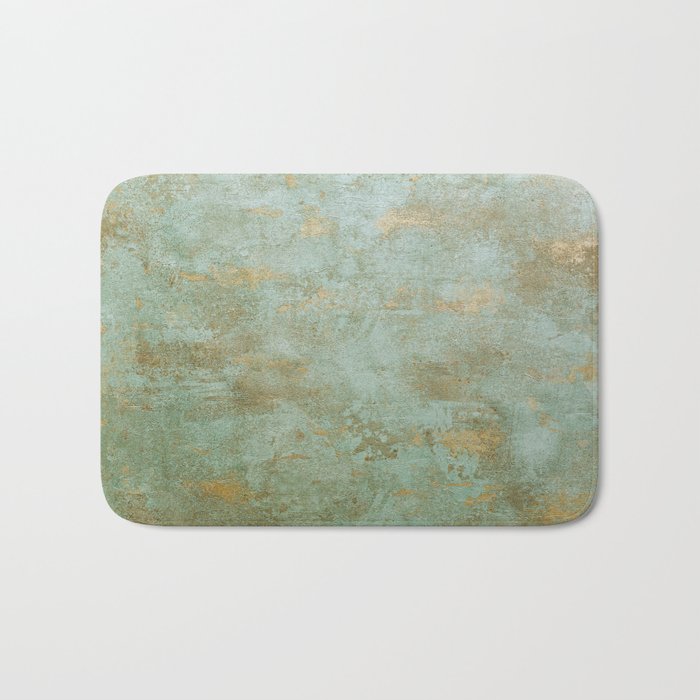This image features a rectangular bath mat with rounded corners, centered against a light gray to white background, leaving about an inch of space around it. The bath mat boasts a metallic appearance, blending green and gold tones with a hint of copper, giving it a worn, scuffed look. Its surface lacks any discernible pattern or text, presenting a random mix of colors and a subtle faded aesthetic. The mat’s metallic sheen and blended colors create a unique, understated design.